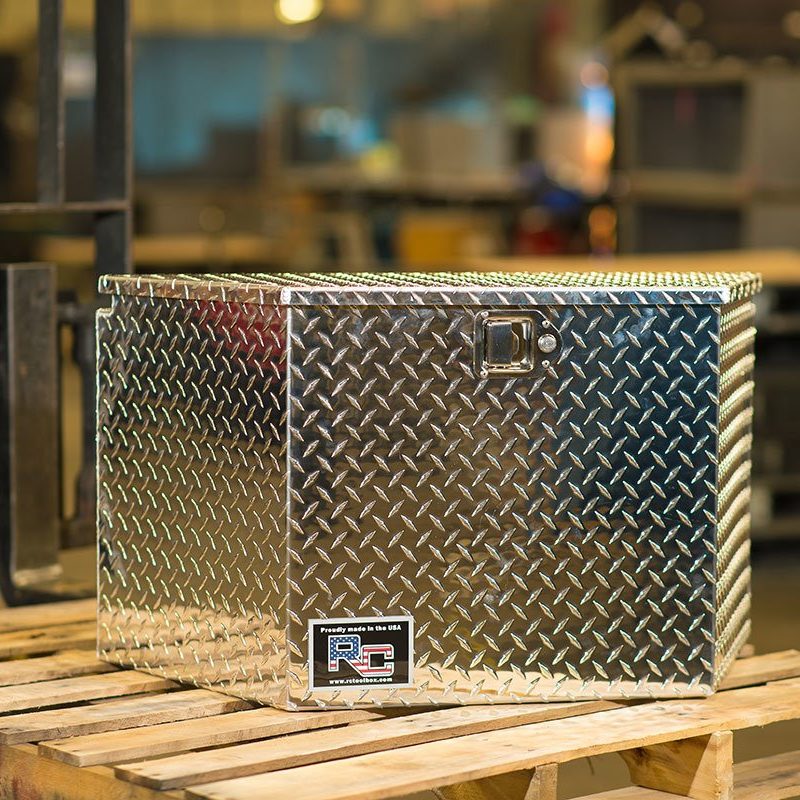This photo shows a silver-coated, possibly metal, lockbox with a reflective surface and a distinctive cross diamond texture. The box has a unique polygonal shape, appearing wide at the front and narrowing towards the sides. The front features a latch at the top center and a sticker on the bottom left, marked with "R.C." in red, blue, and white against a black background with small, unreadable white text above it. The lockbox, which could be a tool chest or storage box, rests on a wooden surface made of horizontal planks with noticeable gaps. In the reflection at the bottom left, the wood surface is visible. The background includes dark shelving or possibly metallic structures to the left, extending out of the frame, and blurry shelves with items and a couple of monitors on the right, suggesting the photo might be taken in a room, possibly a kitchen or a workspace. There's a manufacturer's logo that hints at American origin, with "Proudly made in the USA" and a web address, www.retailbox.com, indicating the item is likely for sale and intended for storing tools or other valuables.